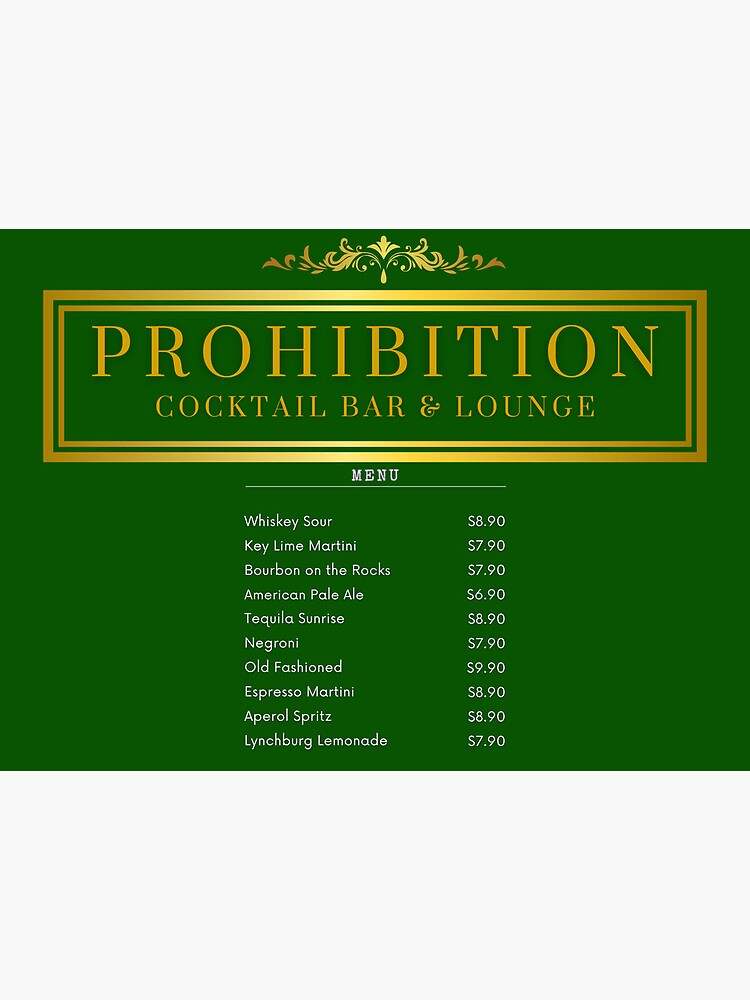The image is a digital menu card for Prohibition Cocktail Bar and Lounge, set against a dark green background. The layout is rectangular in a landscape format. Dominating the top third of the image is a decorative logo featuring the word "PROHIBITION" in large gold letters. Beneath it, in smaller gold font, the words "COCKTAIL BAR & LOUNGE" are displayed. The logo is encased in two gold rectangular borders with an elegant, symmetrical leafy floral design positioned above it.

Below the logo, spanning the bottom two-thirds of the image, is the menu section. The word "MENU" is written in all caps, in white font, with a white line underneath. The menu lists various cocktails and their prices: Whiskey Sour ($8.90), Key Lime Martini ($7.90), Bourbon on the Rocks ($7.90), American Pale Ale ($6.90), Tequila Sunrise ($8.90), Negroni ($7.90), Old Fashioned ($9.90), Espresso Martini ($8.90), Aperol Spritz ($8.90), and Lynchburg Lemonade ($7.90). The prices range from $6.90 to $9.90, presented in a descending order.